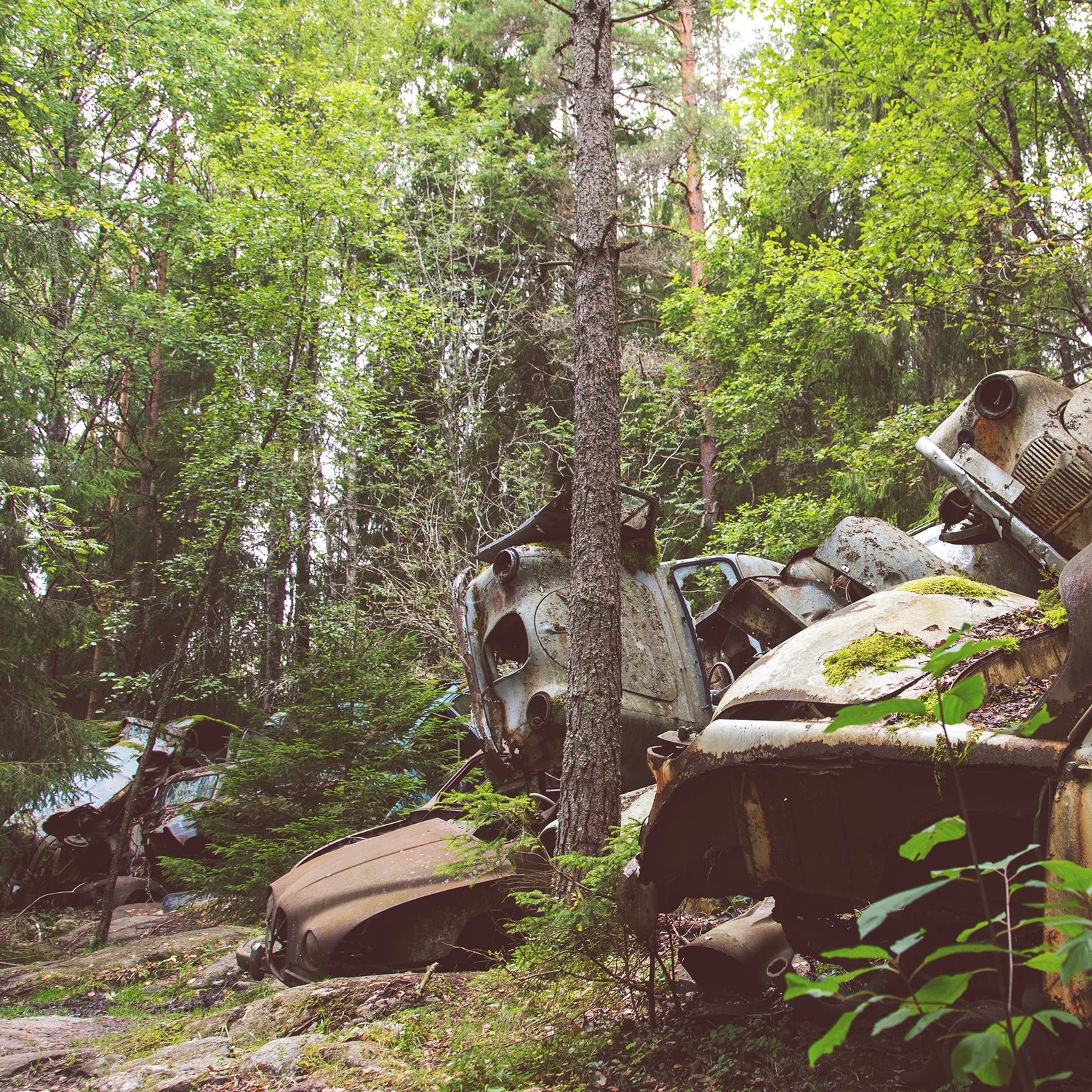In this image, we see an expansive car junkyard situated deep within a dense, green forest. Tall trees, some appearing to hold up the rusted car remains, dominate the backdrop against flashes of a light white sky. Piles of old car bodies, now little more than broken, disintegrating hulks, are stacked on top of each other. To the right, one stack forms a precarious tower resembling dominoes propped up by another rusty car body. Scattered car parts—hoods and other remnants—are strewn across the rocky ground. The scene suggests that the cars have been abandoned here for such a long time that the forest has regrown around them, blending the mechanical detritus with nature’s persistent reclaim.